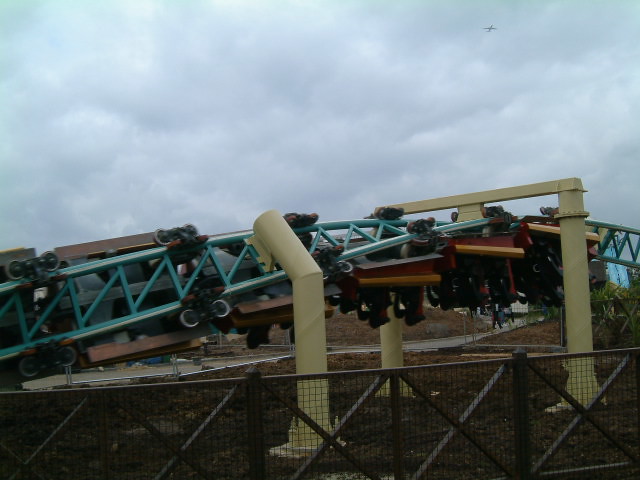The image depicts a dramatic and thrilling outdoor scene at an amusement park on a very cloudy day. The sky is completely obscured by thick, fluffy clouds that vary in shades of gray and white. Dominating the center of the image, a roller coaster twists and turns along light blue rails, supported by sturdy yellow beams. The roller coaster cars, which are red in color, are caught in a heart-stopping moment as they flip upside down. In the foreground, a black fence with thin grates and an X-bar design runs across the lower portion of the image, partially obstructing the view. The ground appears to be a mix of brassy and tan hues, suggesting an open field or a paved area. In the background, a faint structure resembling a blue building is visible, further adding to the amusement park setting. The overall scene is a vivid snapshot capturing the excitement and intensity of a roller coaster ride set against a dramatic sky.